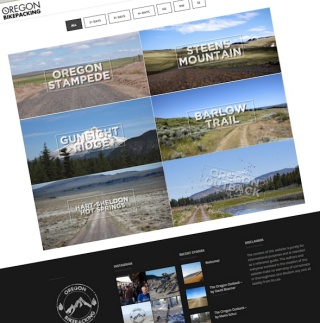This composite image features a series of photographs highlighting several picturesque locations, all set against a clean white background. The following places are depicted: Oregon Stampede, Staines Mountain, Gunsight Road, Bagot Trail, Heart Springs, Heart Sheldon, and Oregon Outback. The images display a palette dominated by green, blue, and black hues, capturing the natural beauty and diverse landscapes of these areas. Notably, Staines Mountain is prominently featured, providing a majestic focal point. Additionally, Heart Sheldon appears multiple times, underlining its significance in the series. The overall composition offers a visually appealing and detailed snapshot of these stunning locations.